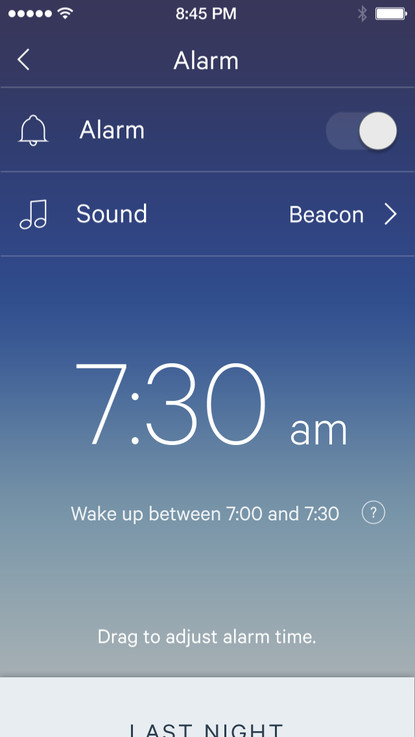The image depicts a cell phone screen with a variety of interface elements displayed against a graduated background. At the top of the screen, signal bars for both phone and Wi-Fi connection are visible, along with the time "8:45 p.m." prominently displayed in the center. On the left side, icons for Bluetooth and a fully charged battery are present.

Below this top section, there is a horizontal line dividing the interface elements. An arrow pointing left is found, with an alarm icon centrally located next to it. Further down, another line separates this section from an alarm toggle switch, which appears ambiguous regarding whether it is on or off.

Continuing downward, a third horizontal line divides this section from another labeled "Sound," which reads "Beacon" next to a right-facing arrow. Beneath yet another line, the text "7:30 a.m. Wake up between 7 and 7:30" is displayed, accompanied by a question mark icon within a circle. The instruction "Drag to adjust alarm time" is placed at the bottom of this section, all set against a background transitioning from dark blue (almost black) at the top to a lighter blue and then off-white near the bottom.

The lowest portion of the screen, set against a white background, features the black text "Last night." The majority of the font used in the interface is white, with the time "7:30" being the most prominent, standing out significantly in size compared to the other text elements.

The color palette of the screen comprises various shades of blue, off-white, white, and black.